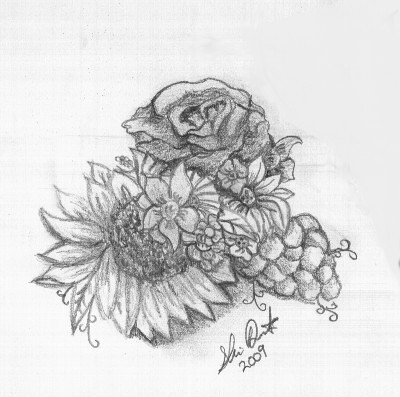This detailed pencil drawing on a white sheet of paper, measuring square, depicts a harmonious still life arrangement combining multiple flowers and fruit. Dominating the composition slightly above center is a meticulously outlined rose, its topmost part outlined while its lower part is richly shaded. To the left below the rose is an intricate daisy, featuring a deeply shaded central bulb and delicately outlined leaves with noticeable vein shading near the center. Adjacent to the daisy on the right is an artistic representation of a bunch of grapes, enhancing the natural element of the drawing. Another daisy, smaller in comparison, occupies the space above and to the left of the grapes with a darker veined pattern and refined leaf details. The central focus also includes a prominent sunflower in the background, adding depth to the cluster. This elaborately shaded piece, revealing a myriad of textures, casts a subtle drop shadow beneath the floral ensemble, further enriching the visual depth. Positioned at the lower center of the drawing, the signature of the artist, possibly "Steve" or "Stu Dent," is inscribed at a 45-degree angle alongside the date "2009," adding a personal touch to this captivating artwork.